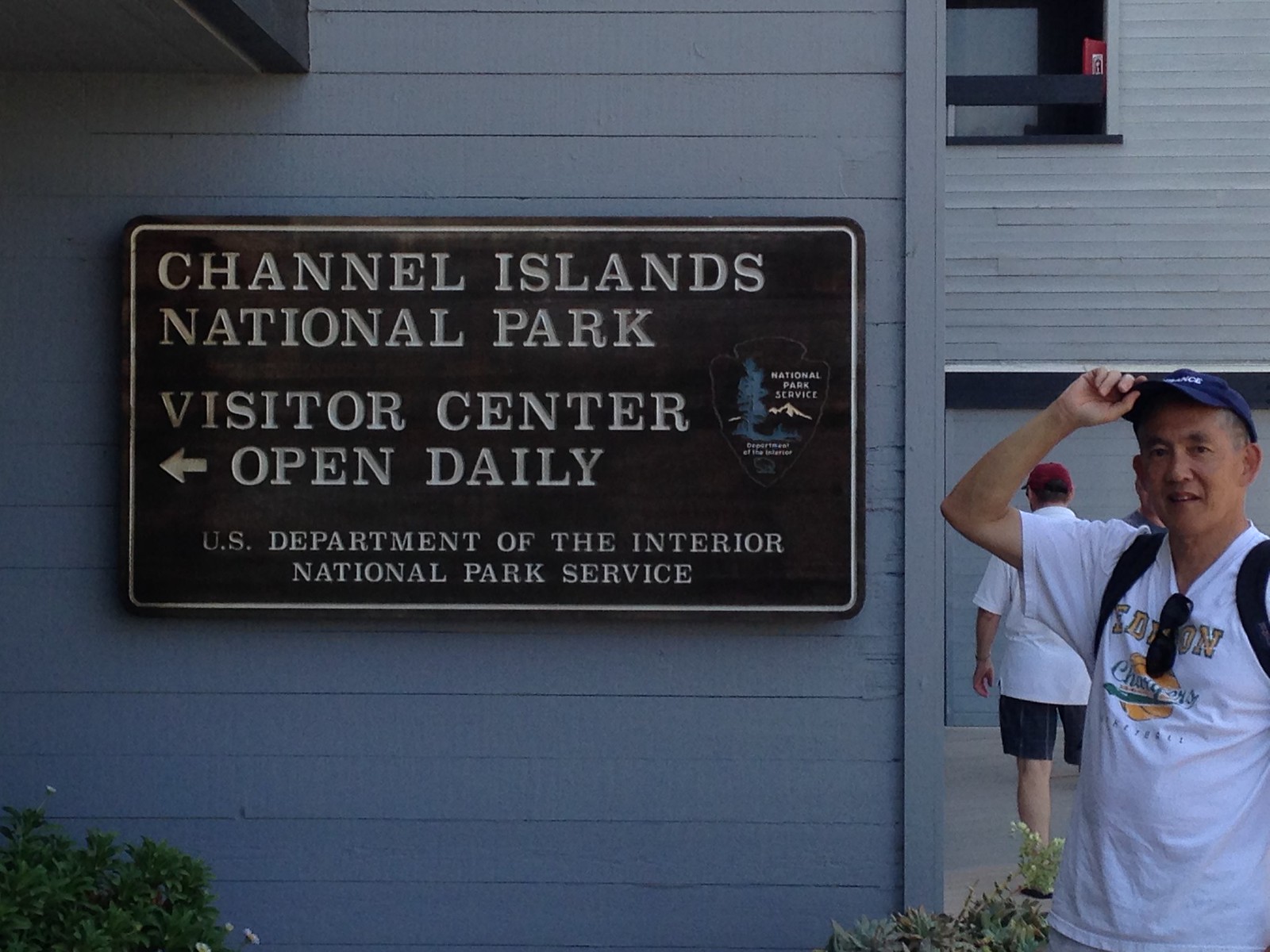The image captures a gray-painted building adorned with a black signboard featuring a white border and white text. The sign reads "Channel Islands National Park, Visitor Center Open Daily, U.S. Department of the Interior, National Park Service." To the right of the sign, a man is posing for the photograph. He is dressed in a short-sleeve white t-shirt with logos on the front, and a pair of black-rimmed, black reflective sunglasses dangle from his collar. He sports a blue baseball cap with white lettering, and the black straps of a backpack rest on his shoulders. The man is holding the tip of his hat with his right hand. Behind him stands another individual facing away from the camera, wearing a white short-sleeve t-shirt, black shorts, and a red baseball cap.